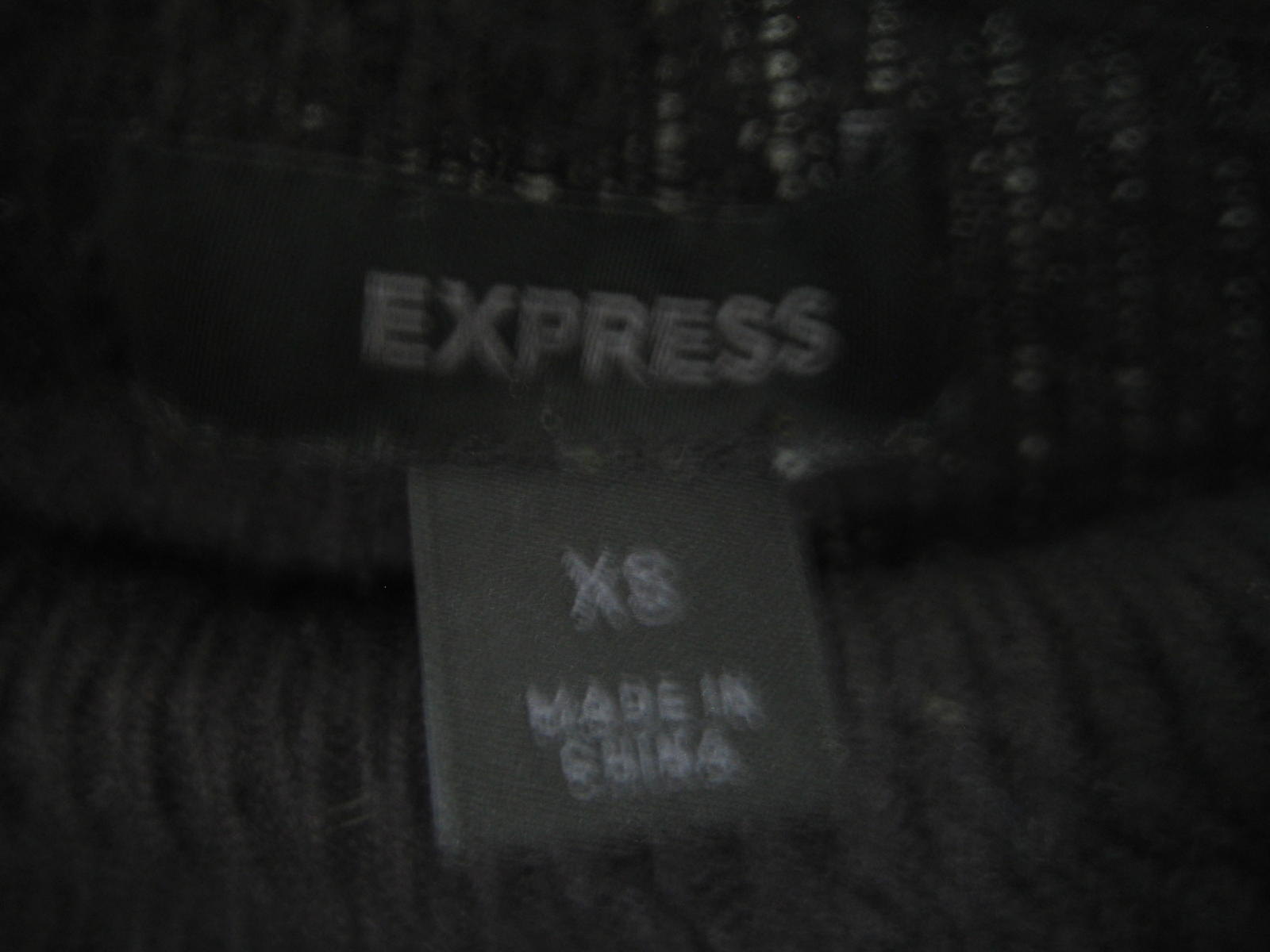This black-and-white photograph, likely taken with a smartphone, offers a close-up view of the inside of a sweater's rolled collar. The sweater fabric appears to be textured, possibly suggesting a cotton or cotton-polyester blend. Dominating the image is a rectangular black tag that reads "EXPRESS" in bold white letters. Below this, a smaller, lighter gray tag with "x8" or "x3"—the exact number is obscured by motion blur—states "MADE IN CHINA." The blurred image hints at the sweater's dark gray or black color, with a pattern of light gray dots on the upper portion transitioning to a solid black lower section, emphasizing the intricate texture and subtle design details of the garment.